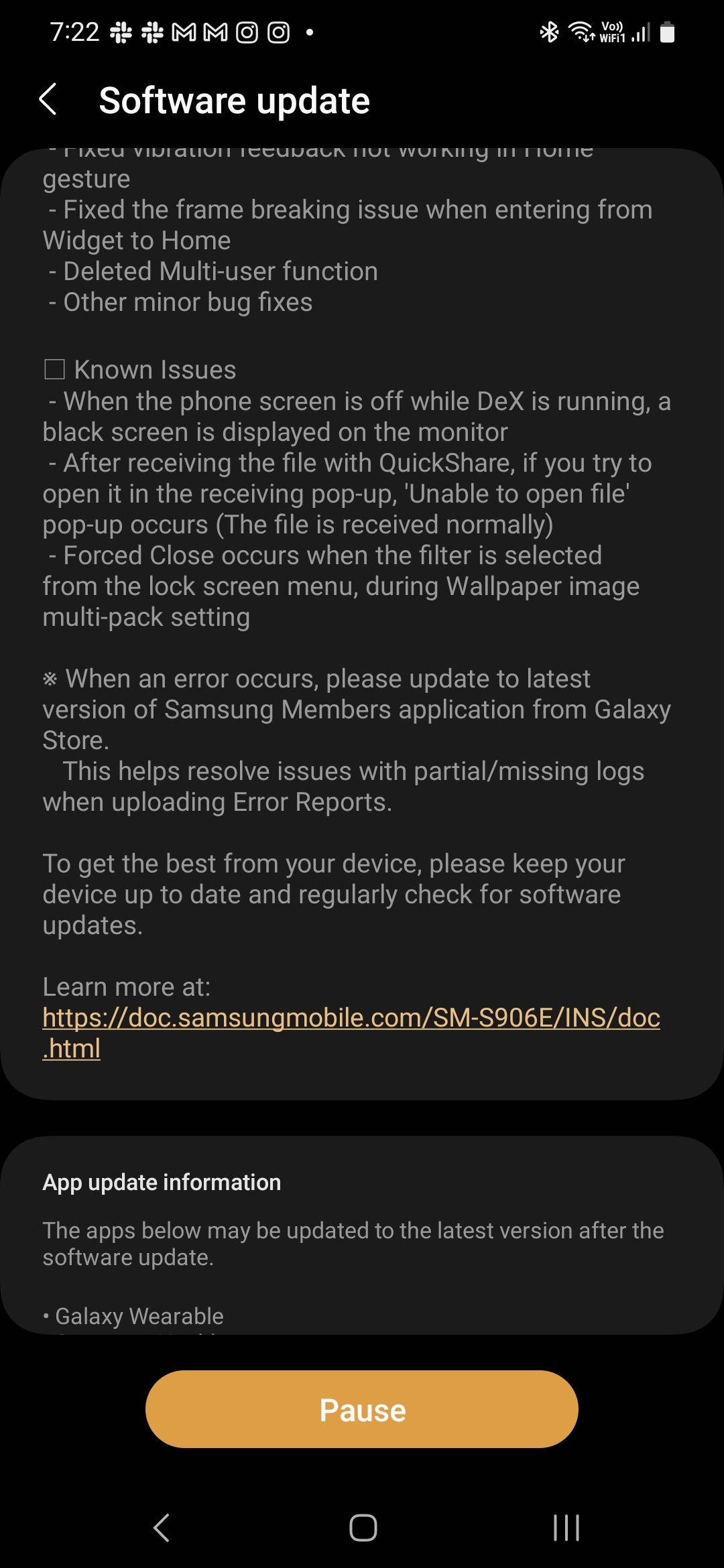A smartphone screen is displayed with a predominantly black background, featuring a software update notification at the top. The text, written in white, informs users about various improvements and bug fixes included in the update. Key points highlighted include: 

- Fix for the frame breaking issue when transitioning from the widget to the home screen
- Removal of the multi-user function
- Other minor bug fixes

Additionally, the update notification lists known issues:

- When the phone screen is off while Samsung DeX is running, a black screen appears on the monitor.
- After receiving a file with Quick Share, attempting to open it results in a "unable to open file" pop-up, though the file is received normally.
- Forced closure occurs when selecting a filter from the lock screen menu during wallpaper image multi-peg setting.

Users are advised to update to the latest version of Samsung Members application from the Galaxy Store to resolve issues with partial or missing logs when uploading error reports. For optimal device performance, the screen encourages keeping the device updated and regularly checking for software updates. 

A URL, written in brown, directs users to learn more: "docs.samsungmobile.com/sms906e/insdoc.html."

Lastly, the update notes indicate that the Galaxy Wearable app may also be updated to the latest version following the software update. An orange pause button is visible at the bottom of the screen.